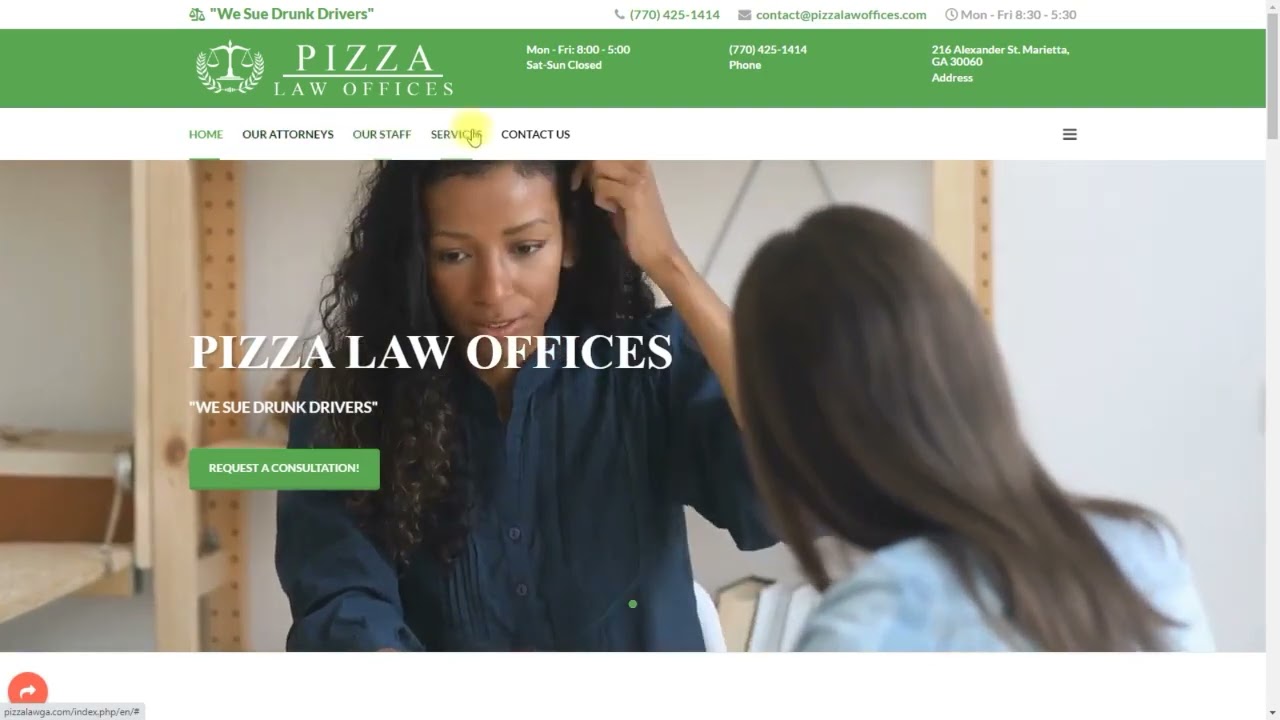The advertisement for PIZZA Law Offices is designed with clear information and distinctive branding. At the very top, a white banner features the firm's tagline in green: "We Sue Drunk Drivers," alongside the phone number "770-425-1414" and the email "contact@pizzalawoffices.com." The hours of operation, "Monday through Friday, 8:30 AM to 5:30 PM," are also listed in gray text.

Below this, a prominent green banner showcases the firm's name, "PIZZA Law Offices," accompanied by an image of a justice scale encircled by laurel leaves. The office hours are reiterated here: "Monday through Friday, 8 AM to 5 PM," with a note that the office is closed on weekends. The phone number is repeated for emphasis, followed by the firm's address: "216 Alexander Street, Marietta, Georgia, 30060."

Underneath this section, a white navigation band provides links to "Home," "Our Attorneys," "Staff," "Services," and "Contact Us," along with an icon of three stacked bars for additional menu options.

The central photograph depicts two women in conversation, both with long hair—the woman on the left has straight hair and is wearing a light blue shirt, while the woman on the right has curly hair and is wearing a blue shirt. Overlaying this image is the firm's name "PIZZA Law Offices" in large white letters, with the tagline "We Sue Drunk Drivers" in smaller text. A green button with white font at the bottom of the image invites potential clients to "Request a Consult."